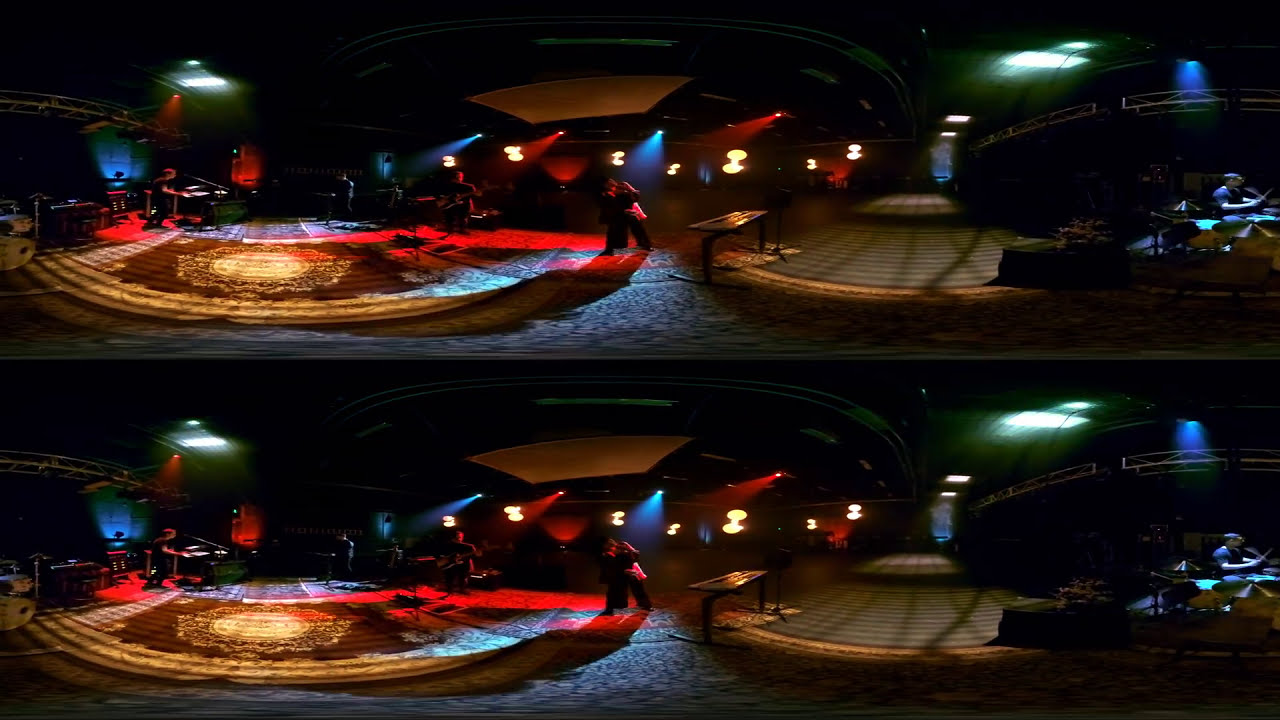The image depicts an indoor music studio with two identical pictures stacked vertically, creating a stereoscopic effect. The rich and intricate stage area is bathed in multiple hues of red, green, and blue studio lighting, contributing to a striking visual atmosphere. On the stage, which is covered by a large red and gold carpet, musicians can be seen engaging with various instruments. Specifically, there are individuals near keyboards and what appears to be a piano. A tan-colored bench is also visible on the stage. The flooring, illuminated by spotlights, exhibits a blend of blue and brownish tones, adding depth to the scene. Bright spotlights are positioned in the upper left and right quadrants of the image, further highlighting the musicians and their instruments. The backdrop of the scene features a dynamic interplay of blue and red lights.